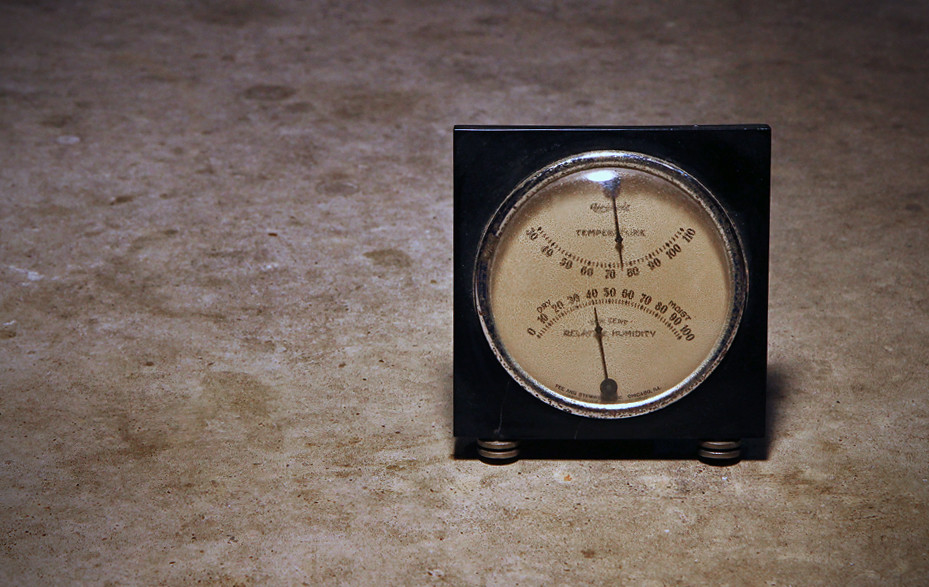The image depicts a metal device housed within a square, black block, resting on a flat, hard surface with a mix of brown, cream, and sandy colors. The device features a round glass face at its center, which is white in color. The face of the device contains two distinct gauges. The upper gauge, labeled "Temperature," displays numbers ranging from 30 to 110, indicating its function as a temperature indicator. The lower gauge, labeled "Relative Humidity," shows numbers from 0 to 100, serving as a humidity indicator. Both gauges are equipped with needles that point to the respective measurements. The precise and detailed design suggests that the device is likely used for monitoring environmental conditions.